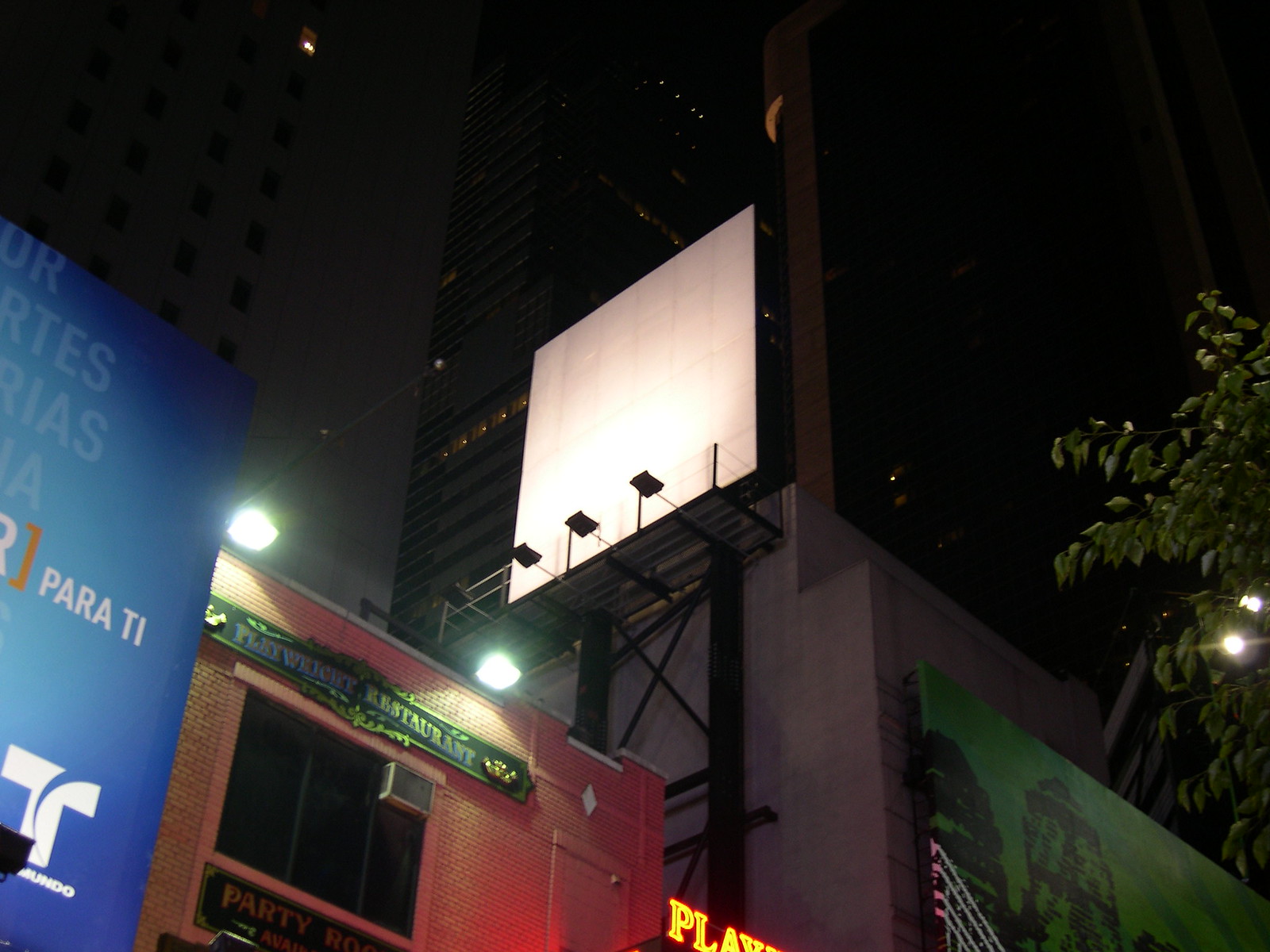This nighttime cityscape photograph captures a towering high-rise building with a strikingly empty white billboard prominently displayed against the dark sky. The brightly lit billboard is held up by a black metal frame and attached to a concrete wall with a glass multi-story building behind it, extending out of the frame. Below the billboard, an orange building with an indiscernible sign and a window with an air conditioner subtly stands out. To the right of this building, a partially visible neon sign reads "Play," possibly part of "Playboy," casting a vivid glow. Adjacent to this is a hunter green wall with an unidentifiable image, while a tree with illuminated leaves occupies the background. On the far left, a blue wall adorned with partially legible white text spelling out "PARA" and "T-T-I" punctuates the scene. The photograph also captures various streetlights and the tops of other buildings, including a red brick building labeled "Playwright Restaurant."